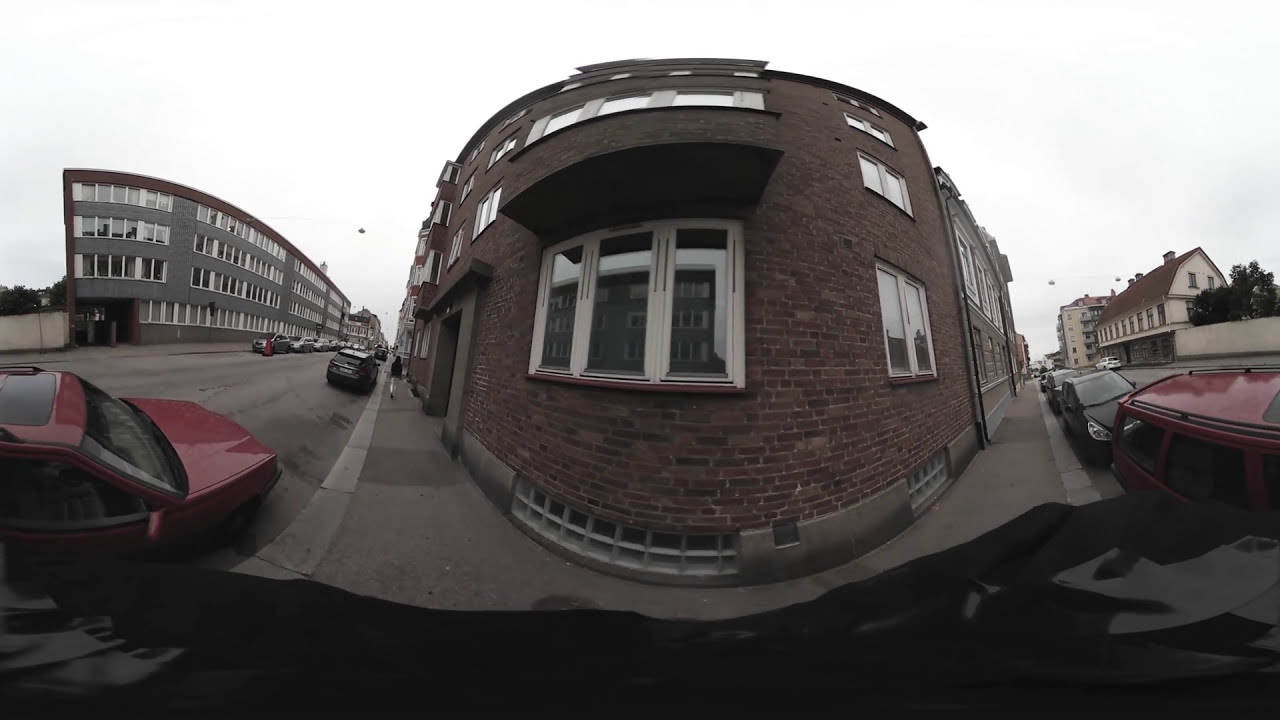The image depicts a panoramic view of a charming urban scene centered around a brick residential building, standing four stories high with numerous windows. The building is flanked by two roads, each lined with cars, notably including a red car and a black car on both sides, positioned in opposite directions. A continuous sidewalk wraps around the entire building, providing a seamless route for pedestrians. The left side of the scene captures a man walking up the sidewalk, next to a row of parked vehicles. The photograph's perspective from the corner where the sidewalks intersect creates a visually engaging panorama, allowing a comprehensive view of both sides of the building and the surrounding streets. To the right, the road is narrow with additional buildings, including larger structures and overhead fixtures that appear to be either lights or traffic signals. The environment includes older structures, contributing to the area's historic feel, under a sky of a whitish hue.